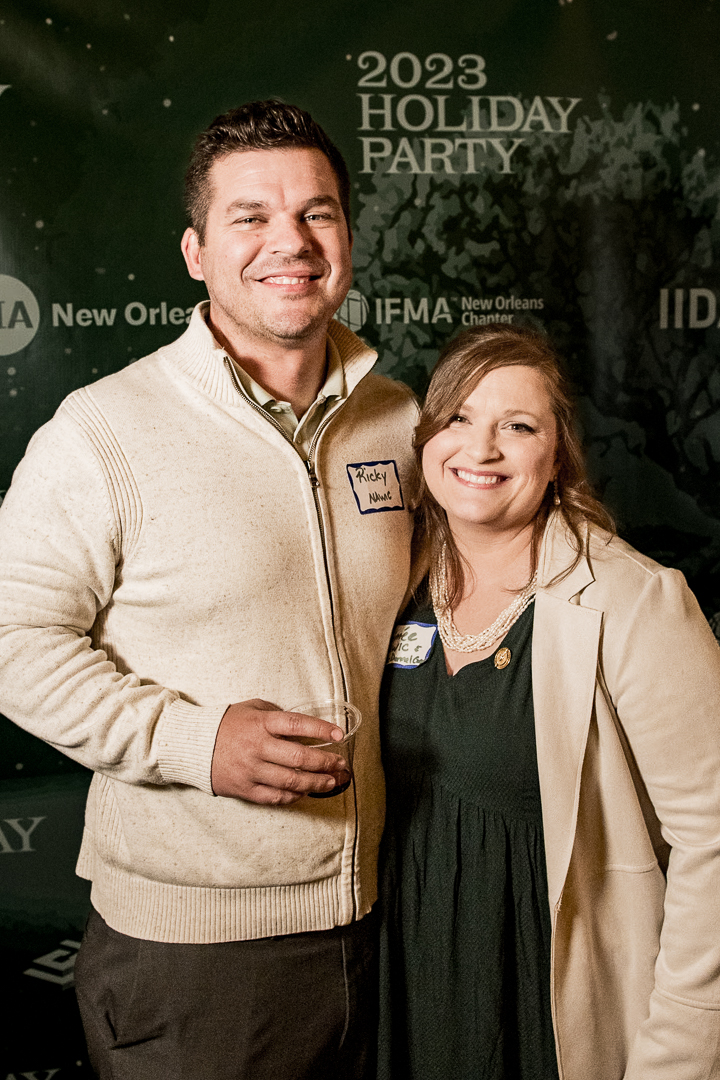In this detailed photograph, two people are posing against a backdrop at a holiday party event. On the left side of the image, there is a tall man with white skin and thin brown hair. He is smiling warmly and is visible from the waist up. He's dressed casually in a zip-up beige-colored sweater paired with dark gray or brown pants. He holds a plastic cup with cola in his hand and has a bit of stubble on his face. To his right stands a woman, who is shorter than the man and is also smiling. She is wearing a dark green dress with a gold button and a light brown or cream-colored trench coat draped over her shoulders. Her long light brown or blonde hair falls gracefully over her shoulders, and she is adorned with a pearl-colored, multi-strand beaded necklace. Both individuals are wearing name tags.

The background is dominated by a large, dark green poster that fills the scene. The poster features a subtle green-shaded floral pattern in the top right corner and numerous repeating logos scattered across it. Prominently written in light green font near the top, just to the right of the center, are the words "2023 Holiday Party." Below this, there is also a round logo accompanied by the text "IFMA New Orleans Chapter," further emphasizing the event's festive theme and setting.